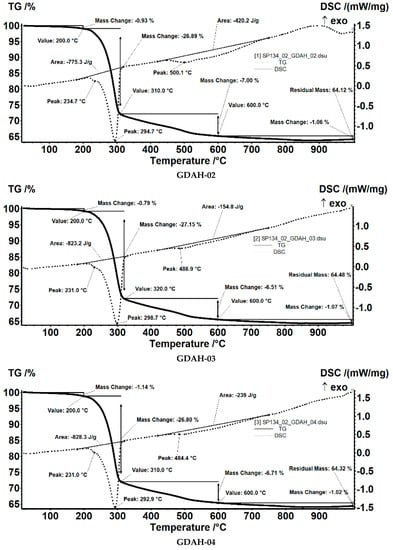The image features a vertical arrangement of three black-and-white graphs, each measuring various parameters related to temperature in degrees Celsius on the x-axis. On the right axis of each graph, the metric "Tg percentage" ranges from 65 to 100. The left axis displays "DSC/MW/MG," with the scale varying slightly among the graphs: the top two ranging from -1 to 1.5, and the bottom one from -1.5 to 1.5. The graphs are labeled respectively as GDH 0.2 (top), GDH 0.3 (middle), and GDH 0.4 (bottom). Despite numerous notations and printings inside the graphs, the text remains illegible due to poor image quality. These graphs likely pertain to some thermodynamic or material property analysis, possibly within the fields of physics or chemistry.